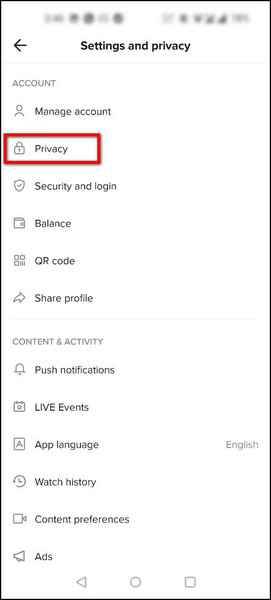This image appears to be a screenshot from a mobile phone. The screenshot itself is a thin, rectangular shape with a predominantly white background, bordered by a thin black line. At the very top, there are a series of blurred-out icons, likely the typical status bar icons seen on most phones.

Below these icons, there is a navigation arrow pointing left, next to the words "Settings and Privacy." The content is divided into sections with various options listed under each.

The first section includes:
- Account
- Manage Accounts
- Privacy (highlighted with a red outline)
- Security and Login
- Balance
- QR Code
- Share Profile

The second section, labeled "Content and Activity," includes:
- Push Notifications
- Live Events (with "Live" capitalized)
- App Language (currently set to English)
- Watch History
- Content Preferences
- Ads

Each option features a small icon to its left. At the very bottom of the image, there are three navigation icons: a left arrow, a circle, and a square.